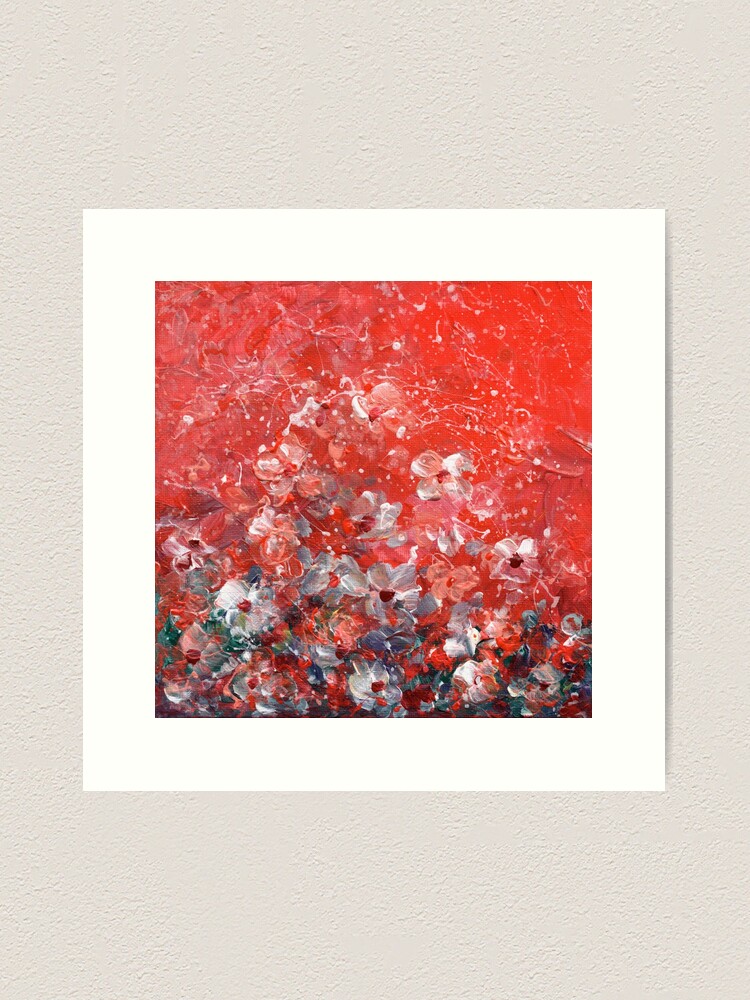This descriptive caption consolidates the details from multiple perspectives into a cohesive narrative:

Hanging on a cream-colored, textured wall is a captivating painting encased in a simple, white frame. The painting, which seems to be a printed reproduction on canvas rather than a hand-painted original, features a striking red background with a prominent motif of white flowers, vaguely resembling dogwood blossoms. The flowers are detailed with red centers and are accompanied by hints of green, suggesting leaves. Adding to the painting's depth are white splatters that create a textured effect, and a few flowers in blues and grays, giving the piece a hectic, abstract quality. Despite its abstract and somewhat smudged appearance, the main subject of the painting remains vivid—an array of white and pink flowers set against a rich, red backdrop. The overall composition is square in shape, complementing the neat, framed presentation on the wall.